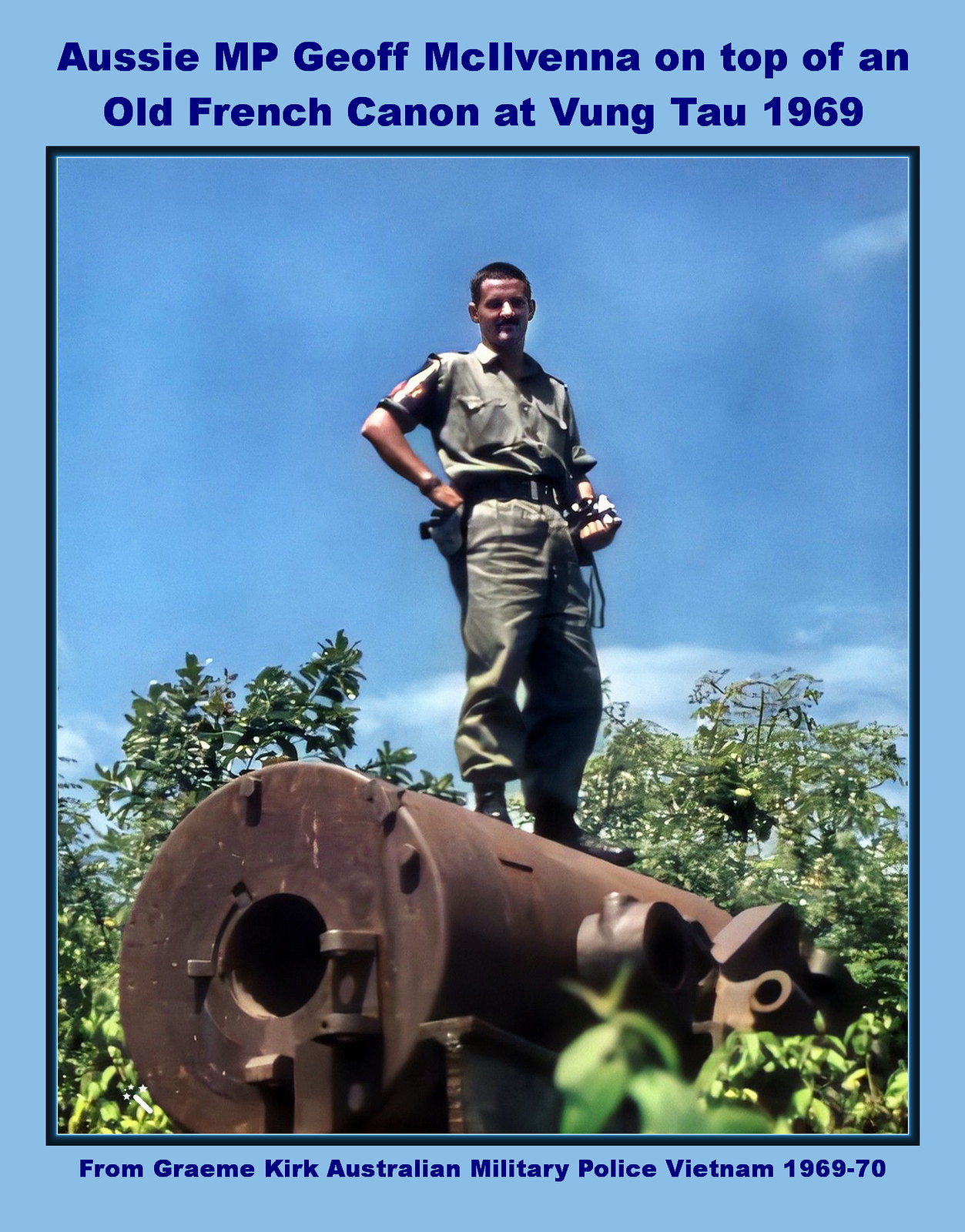The photograph, framed in a muted light blue border, depicts a soldier standing on top of an old, rusted French cannon at Vung Tau in 1969. The man, identified by the inscription above the photograph as Aussie MP Jeff McClevenna, wears a green army shirt, green pants, and sturdy boots. He stands confidently, one hand resting on his shoulder, looking down at the viewer. The cannon, with a bronze coloration due to rust, is surrounded by lush vegetation and trees, with a mostly clear blue sky dotted with a few mild clouds in the background. At the bottom, the text reveals that this image is credited to Graham Kirk of the Australian Military Police, Vietnam 1969-1970, with a note that reads, "Does this happen here?"